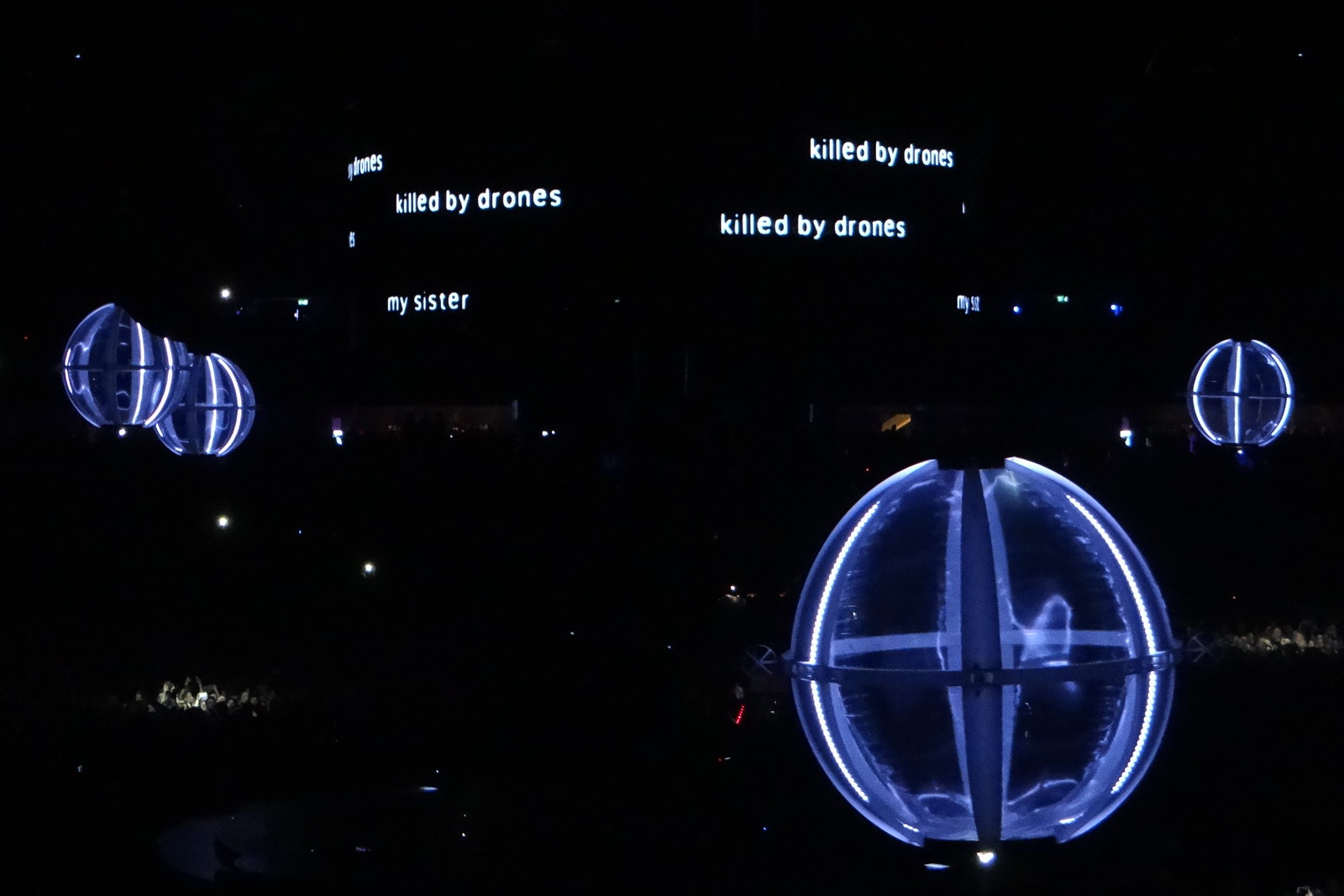This image appears to be a digitally enhanced or AI-generated photograph of an intense and captivating light show set against a dark background. Dominating the scene are four large, hollow spherical structures, each illuminated with blue light inside and bordered by white lines that run top to bottom like latitude lines, giving them an ethereal glow. The tops and bottoms of these structures are noticeably darker. Suspended in the sky within these structures, multiple lines of text repeat the words "killed by drones" in an off whitish-blue hue, contributing to a haunting atmosphere. Additional text saying "my sister" can also be faintly seen towards the bottom left. 

In the lower part of the image, despite the darkness, details emerge when zoomed in. On the bottom left, a group of people with raised arms appear to be enjoying the spectacle, some holding cameras to capture the moment. On the right side, another group is partially illuminated by ceiling lights, creating a stark contrast against the dark surroundings. The entire scene evokes a sense of otherworldliness, with hints of a space or sci-fi theme, possibly suggested by the depiction of stars or floating rocks in the background.